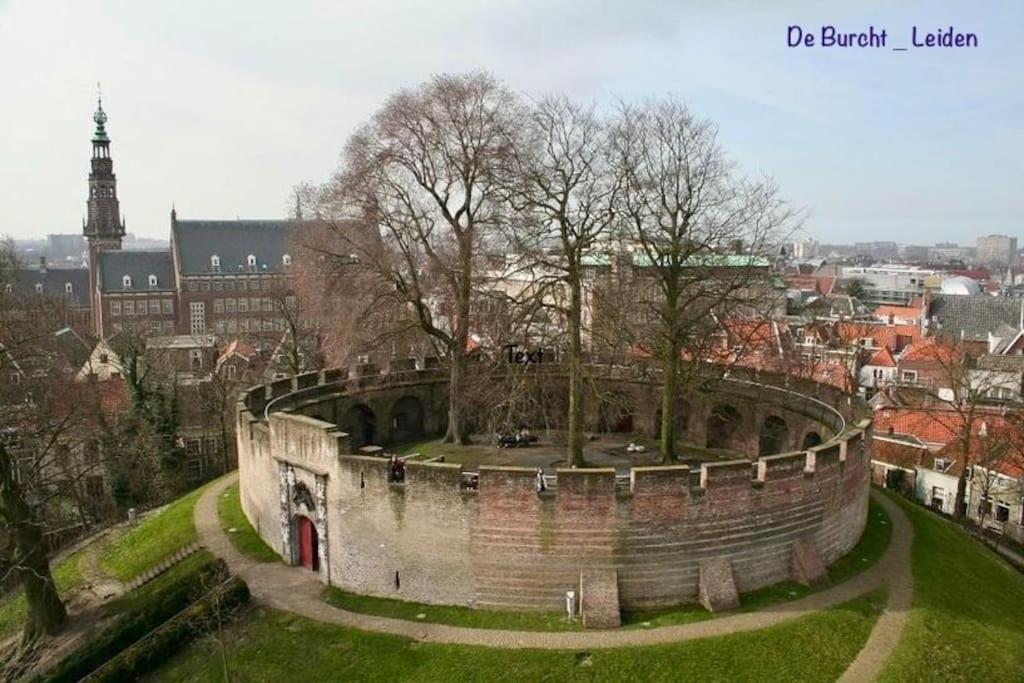This is an aerial photograph capturing a unique park-like setting on a hill, centered around a circular stone structure known as "De Burcht – Leiden." The structure features a roofless, moss-covered stone wall with prominent red doors and an inscription visible on the upper part. Inside this circular fortification are three tall, leafless trees. Surrounding it is a lush expanse of green grass, with a sidewalk encircling the entire structure. A path extends from the lower right corner of the image, while a set of steps is visible on the left.

In the background, the photograph showcases a European cityscape with a variety of multi-story buildings. A notable edifice is a church with a steeple, distinguishable by its traditional architecture. The roofs of the buildings in the background are predominantly black, red, and a light green, contributing to the picturesque skyline under a slightly overcast blue sky. The image also includes white buildings with red roofs and a seven-story building with a green top nestled among other residential and official-looking structures, creating a diverse urban vista.